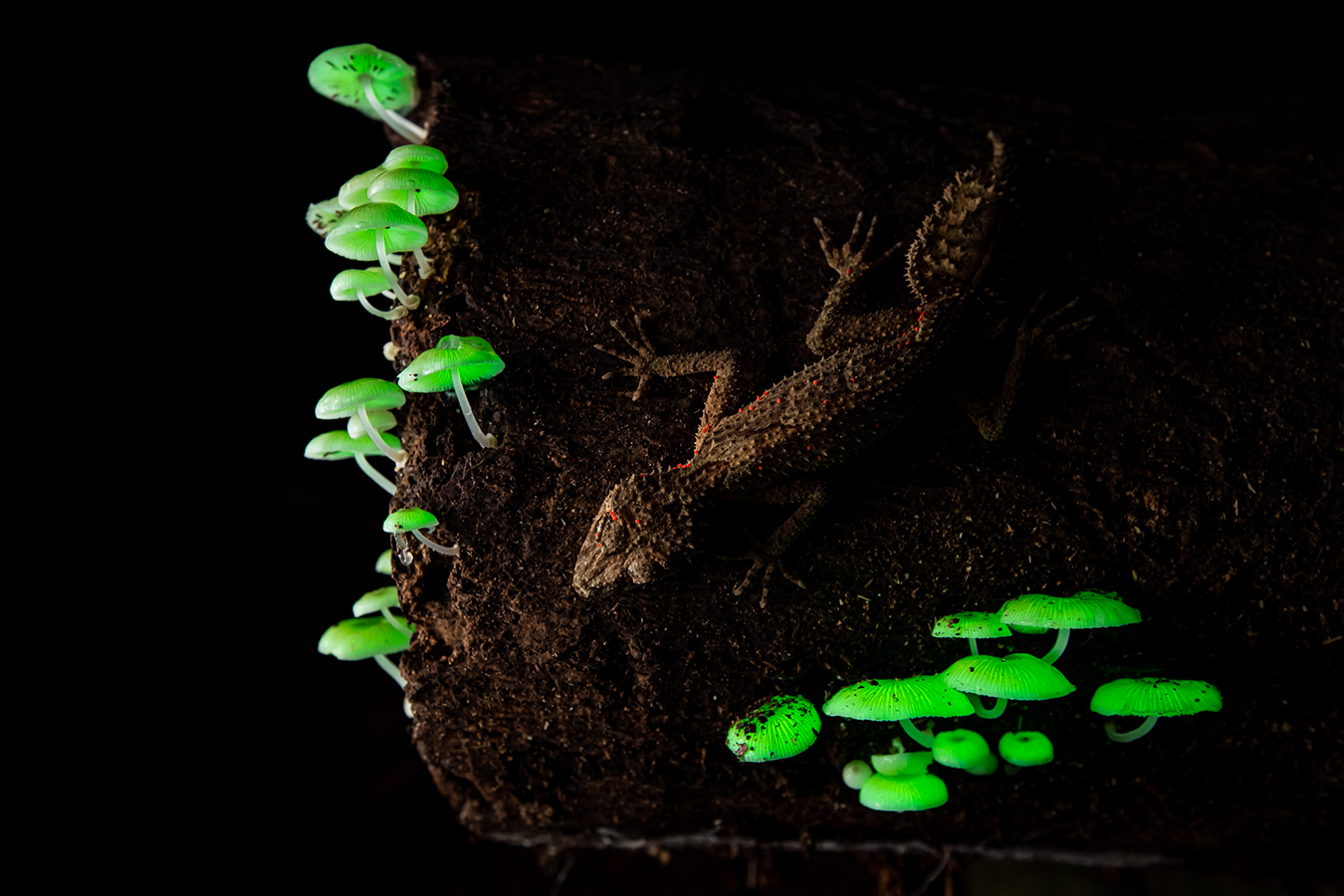The image captures a close-up, landscape-oriented scene at night, possibly under ultraviolet lighting, featuring what appears to be a gecko or salamander lying on a dark brown growth medium that occupies the majority of the frame—from the extreme right to the middle left. The gecko is well-camouflaged with its dark color blending seamlessly into the medium, yet it is distinguishable by bright red spots running along its spine. The creature has a plump body, visible from the top, showcasing four legs with five digits each, and a notably flat, wide tail adorned with spikes, akin to a spiky leaf. Surrounding the gecko, sprouting from the brown earth, are numerous small, neon green mushrooms, their caps glowing luminescently, adding a vivid contrast to the scene and highlighting the textured, spiky appearance of the gecko.